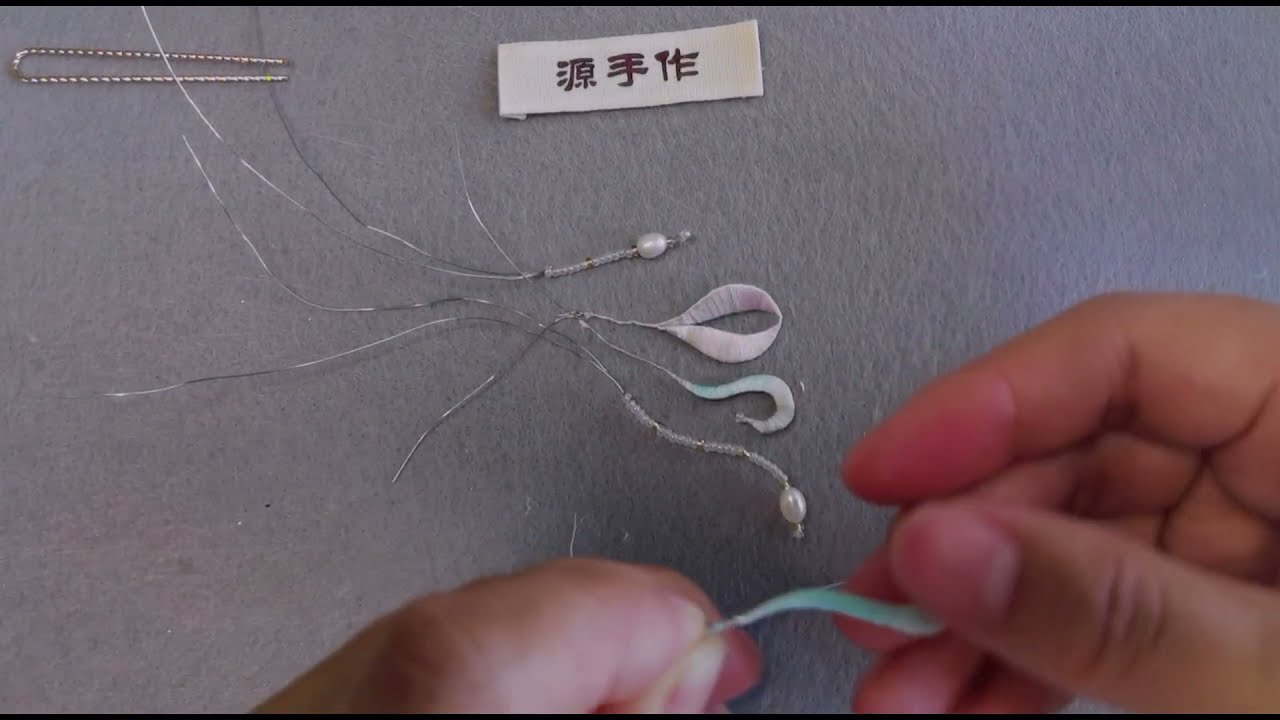In this indoor craft scene set against a gray, fabric-like background, the image showcases two hands at the bottom right, holding a green wire wrapped in green fabric. At the top of the image, there is a small white rectangular paper with three Chinese characters on it. Centrally positioned, several silver wires are present with one end featuring tiny beads and larger white beads. Additionally, metal wires and hooks with small loops of fabric are visible. A pink ribbon is also attached to one of the wires. The image includes distinct colors such as silver, white, green, brown, and tan, contributing to its artistic and detailed composition.